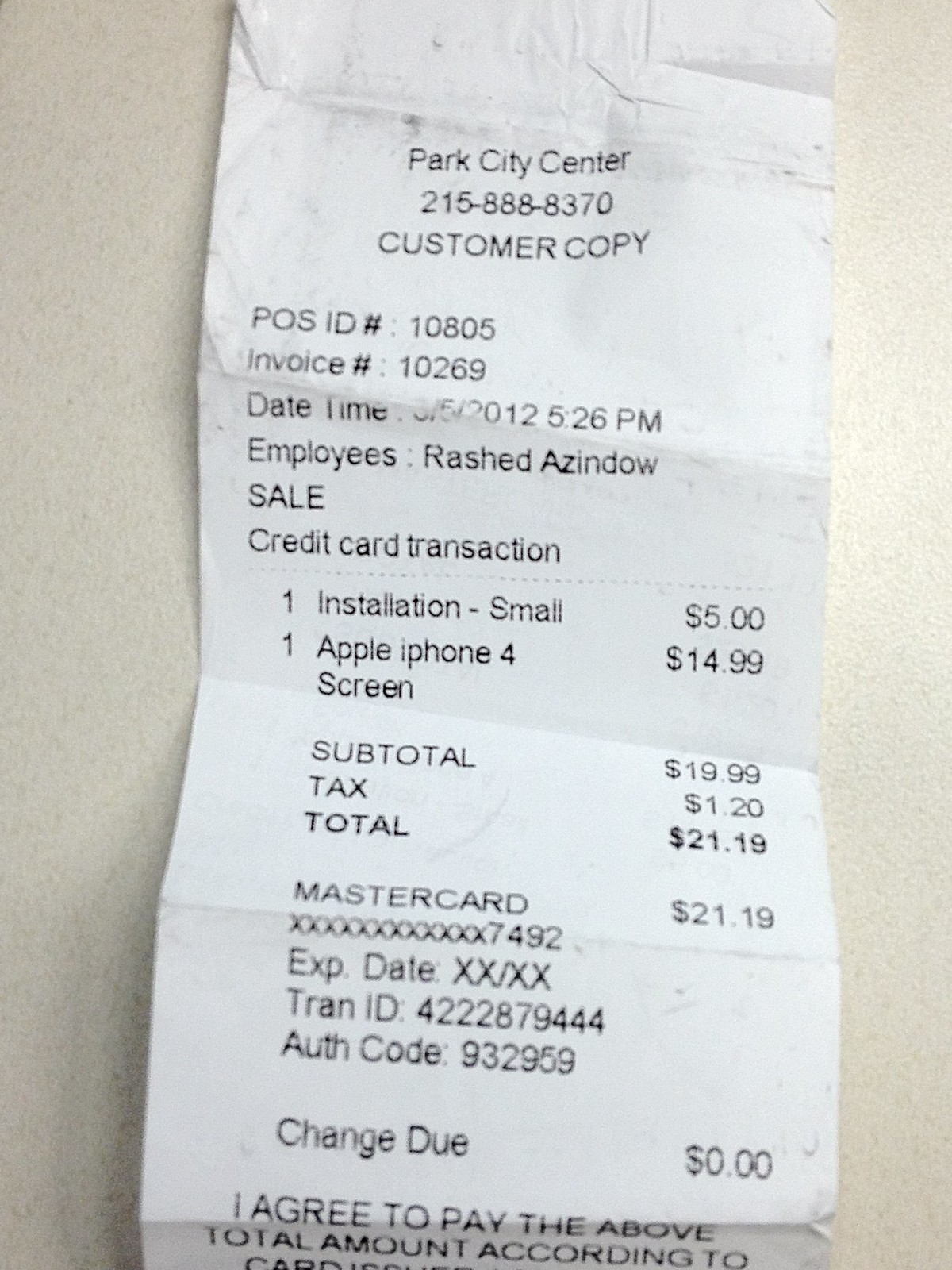This photograph captures a crumpled and wrinkled rectangular paper receipt placed vertically on a white tabletop. At the top of the receipt, printed in black letters, it reads "Park City Center" followed by the phone number 215-888-8370 and the label "Customer Copy." Below that, the receipt lists "POS ID: 10805" and "Invoice Number: 10269," along with the date and time "03/05/20 12:05:26 PM." The employee's name is "Rashad Azendow." The transaction detailed is a credit card sale that includes one "Installation, small" costing $5.00 and one "Apple iPhone 4 screen" priced at $14.99, leading to a subtotal of $19.99. After adding tax of $1.20, the total amount comes to $21.19. The payment was made using a MasterCard with the last four digits 7492, recorded under "Authorization Code: 932959." The receipt concludes with a truncated agreeing-to-pay statement based on the card details.